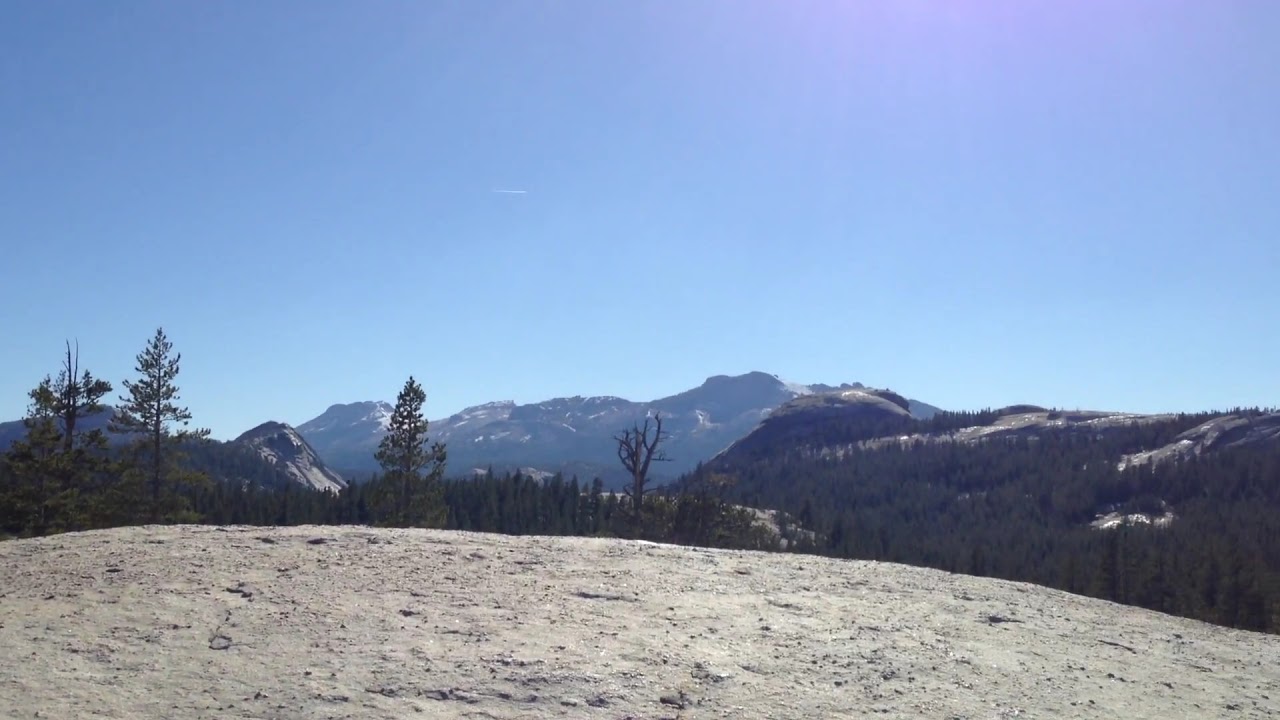This is a detailed photograph capturing a serene, untouched natural landscape without any sign of human presence. The foreground features a rounded expanse of tan-colored sand mixed with pebbles, perhaps situated atop a hill or mountain summit. Dominating the edge of the sandy area are several trees, with two prominent ones on the left, followed by spaced-out clusters of trees, including one that is completely void of leaves. The middle ground reveals a large pine tree accompanied by a few other trees, set against a thin line of trees that stretch towards the horizon. In the background, rolling hills and towering mountains are visible, some with snow-capped peaks. The right side of the image showcases a dense, green forested area. The sky occupies the top half of the image, virtually cloudless and brilliantly clear, with the sun shining down brightly from the top left, illuminating the entire landscape below. This vivid depiction offers a refreshing view of nature in its purest form.